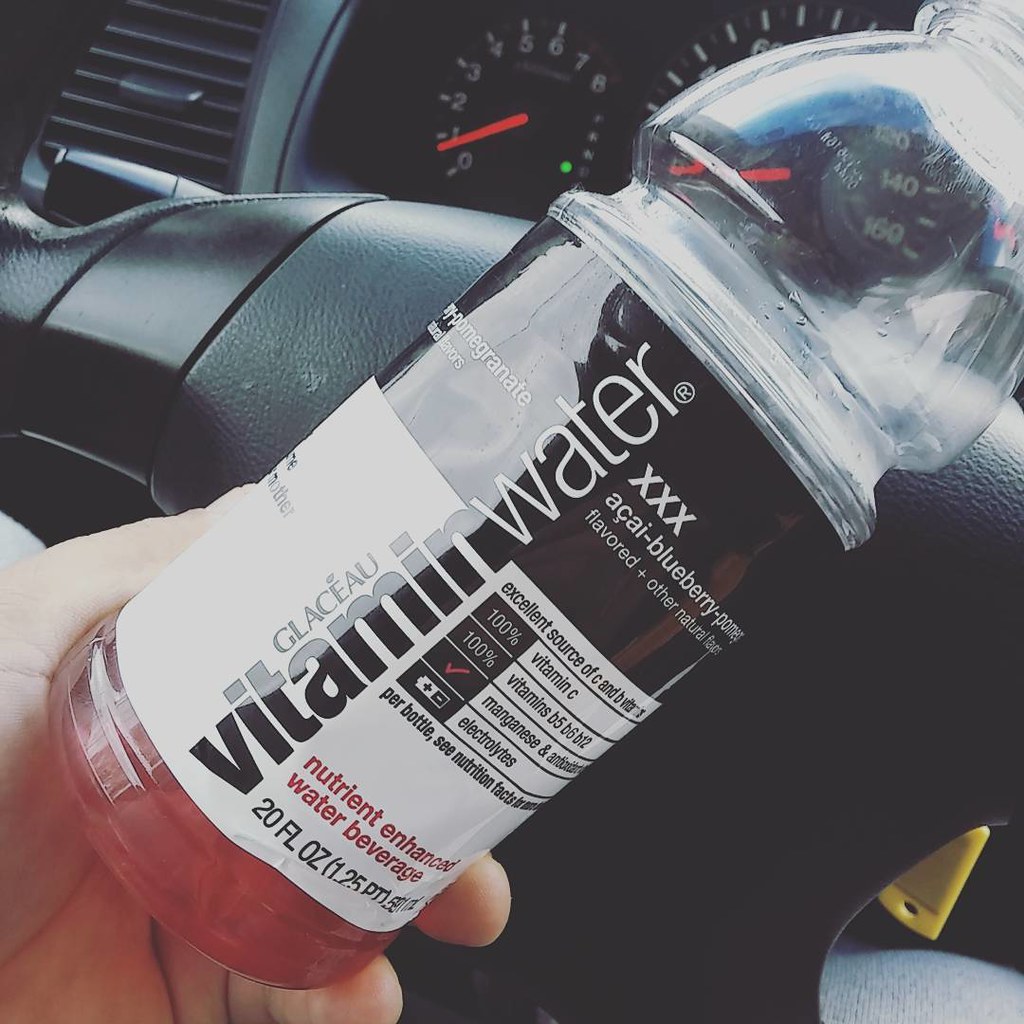Here we have a detailed close-up image of a person seated inside a car. The black dashboard with its curvature prominently frames the scene, and the tachometer is visible in the background. The individual is holding a partially empty bottle of nutrient-enhanced Vitamin Water in their left hand, near the steering wheel. The label on the bottle, displaying an acai, blueberry, and pomegranate flavor, highlights nutritional claims such as 100% of the daily recommended intake of Vitamin C, B vitamins, and manganese, along with electrolytes. The bottle has just enough liquid to cover the bottom. Natural light filters through the windshield, illuminating the bottle and casting subtle reflections on the dashboard.